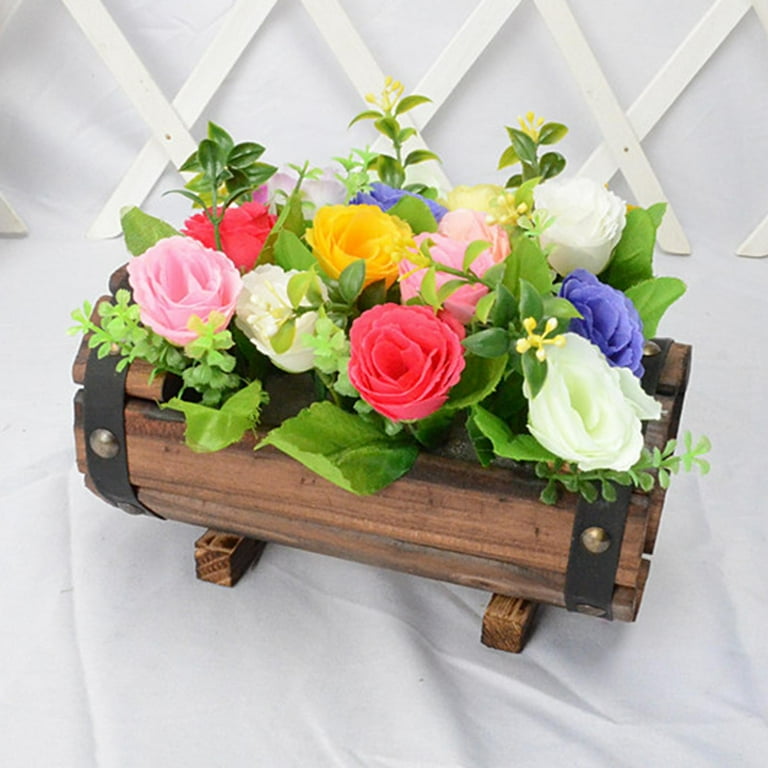The image depicts a vibrant, detailed floral arrangement planted in a small, unique wooden container. This container, resembling a rustic log, is crafted from thin wooden planks and reinforced with two metal straps, possibly leather, held together by brass rivets. It rests on two petite wooden legs. The arrangement features an array of beautiful, presumably live flowers in hues of hot pink, regular pink, white, red, yellow, violet, purple, and blue, all surrounded by lush green leaves. The flowers, which resemble roses, are uniformly sized in bloom, adding to the colorful display. In the background, a white lattice structure, resembling a picket fence with an X-shaped design, provides a quaint backdrop against a white sheet or tablecloth, enhancing the overall aesthetic of the display. The photograph, likely taken indoors, exudes a picturesque and somewhat whimsical charm.